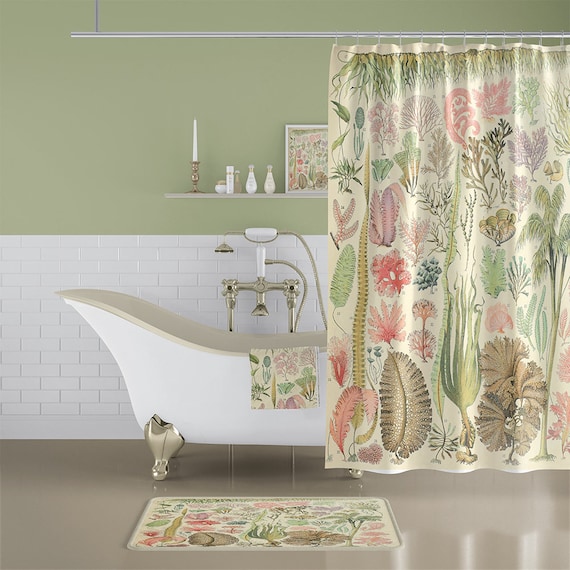This photograph captures a uniquely styled, early 20th-century renovated bathroom. The upper part of the wall is painted in a light moss green, while the lower half is clad in white ceramic tile, giving the space a distinct two-toned appearance. A standalone white ceramic bathtub with a boat-like shape prominently occupies the scene, elevated on four shiny silver legs, matching the detachable, also shiny, silver shower head and fixtures.

Above the bathtub, a shelf on the green portion of the wall holds various items, including an unlit tapered candle in a shiny holder, small bottles of lotion, shampoos, and soaps, as well as a small painting that mirrors the pattern found elsewhere in the room. The scene is tied together by a nature-themed shower curtain hanging from a ceiling-mounted silver rod. The curtain has a beige background decorated with green and brown plants, grasses, trees, and interspersed red flowers. This pattern is consistently echoed across a matching floor mat and an adjacent towel draped over the edge of the tub. Complementing the vintage ambiance, the floor is made of a glossy dark brownish-grey material, adding a touch of modern elegance to the historical aesthetic.